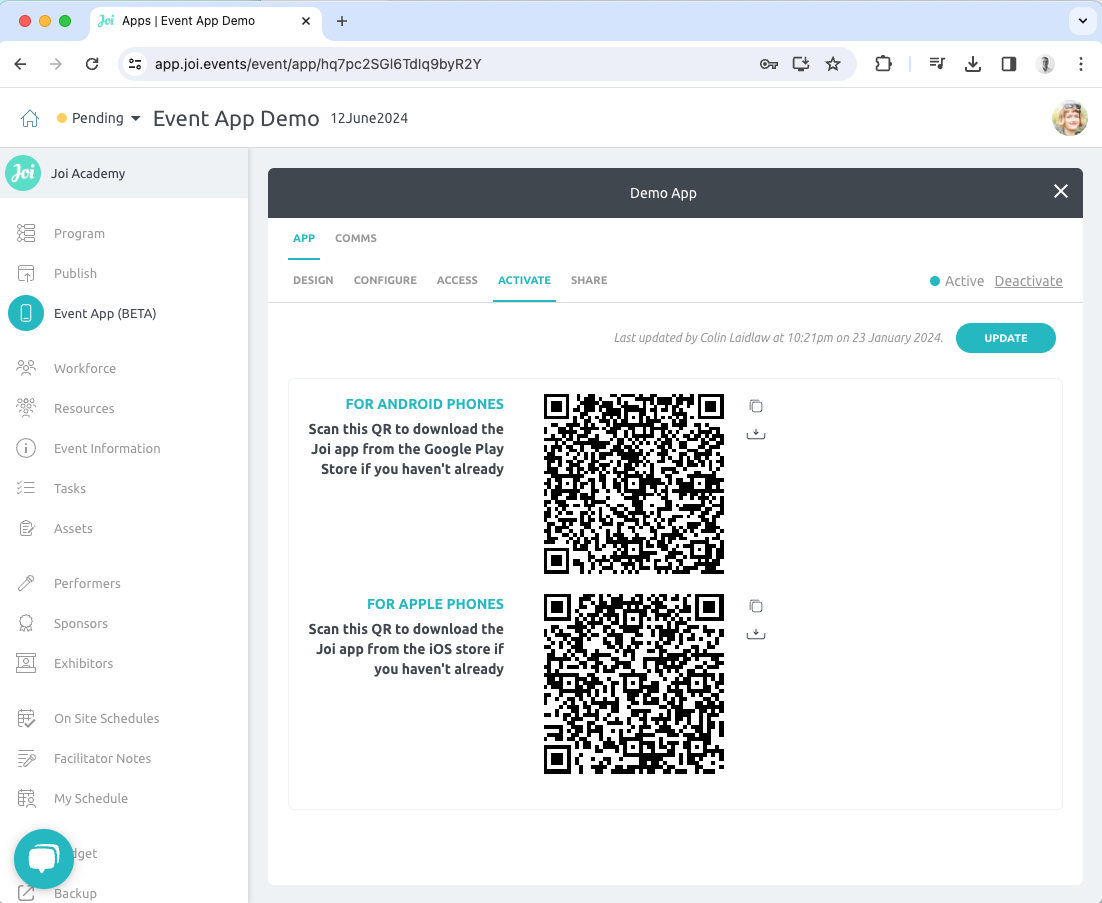Here is a detailed, cleaned-up caption for the provided image description:

---

This image captures a screenshot of a web page within a browser window set against a very light blue background. The browser has one open tab, which is gray and titled "Apps Event App Demo." The web address displayed reads "app.joi.events/events/app" followed by a string of letters and numbers. On the left side of the page, there is a label "Pending," and centered below in prominent gray font, the text "Event App Demo" appears. The date "12 June 2024" is shown in a slightly smaller font beneath this title. On the far right side of the page, there is a circular profile photo that seems to depict a white man, though it is too small to discern any details clearly.

To the left, a sidebar header reads "JOI Academy," featuring the Academy's logo—a circular emblem in aquamarine blue with "JOI" inscribed in white. The sidebar lists various menu items, such as "Program," "Publish," "Event App (beta)," "Workforce," "Resources," and more. This list extends quite long.

Occupying approximately three-quarters of the page, against a white background, is a top border in dark gray, almost black, with the text "Demo App" written in white. Below this, there is a menu bar with items labeled "Design," "Configure," "Access" and the currently selected "Activate" written in blue. To the right of this menu bar is a "Share" button.

Centered on the page are two large QR codes, one above the other. The top QR code is labeled in blue font as "For Android Phones," and the bottom QR code is labeled "For Apple Phones." Each description advises scanning the corresponding QR code to download the JOI app from Google Play for Android devices or the iOS App Store for Apple devices.

---